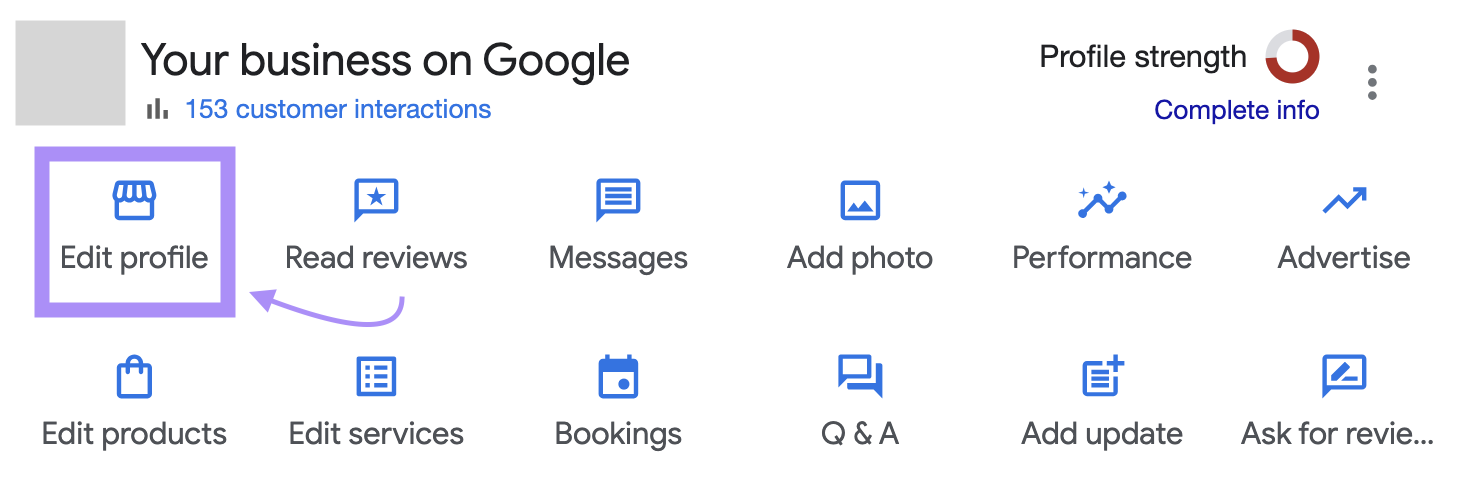Top left of the image features a gray square. Below that, there is a blue section labeled "Your Business on Google" showing 150 customer interactions. The image includes a straight blue circle with text that reads "Complete Info," followed by a blue-bordered button that says "Edit Profile."

Moving down, there is a section encouraging users to read reviews, with an arrow pointing to various action items such as "Messages," "Add Photo," "Performance," "Advertise," "Edit Products," "Edit Services," "Bookings," "Q&A," and "Updates."

The image appears to be a snapshot of a user interface for managing a business profile on Google, showing essential features and actionable options for enhancing the profile and engaging with customers. It highlights the total number of customer interactions (150) and provides easy access to editing information, interacting with messages, and updating various business details.